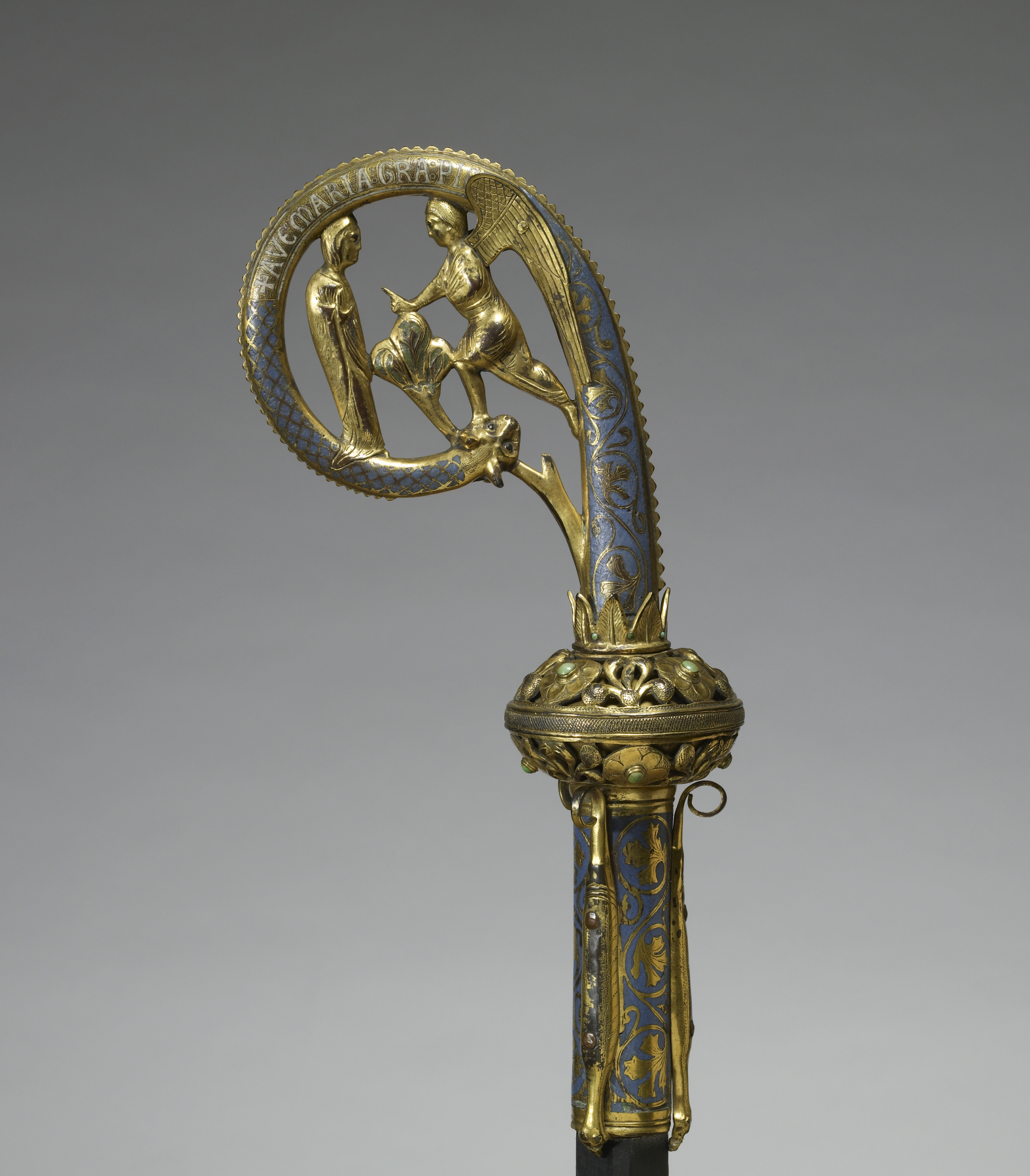The image depicts the intricately designed handle of a walking stick or possibly a staff, crafted from metal with lavish gold and silver or iron elements. The handle showcases a highly detailed and ornate design, featuring a looping structure adorned with two figures—an angel and a human. The angel appears to be pointing hastily towards the human, possibly imparting a message of piety. Beneath the loop, detailed engravings in what seems to be Latin text, although partially worn and illegible, include phrases like "Pave Maria Graup." The central part of the handle boasts a protruding, flowery motif resembling a clover or fleur-de-lis, accentuated with lavender touches. Additionally, there is an animal figure, possibly a dragon or dragon-dog hybrid, wrapping around the staff. The overall aesthetic is lavish and ornate, contributing to the object's bougie appearance. The artifact is set against a gray backdrop, further emphasizing its historical and artistic significance.